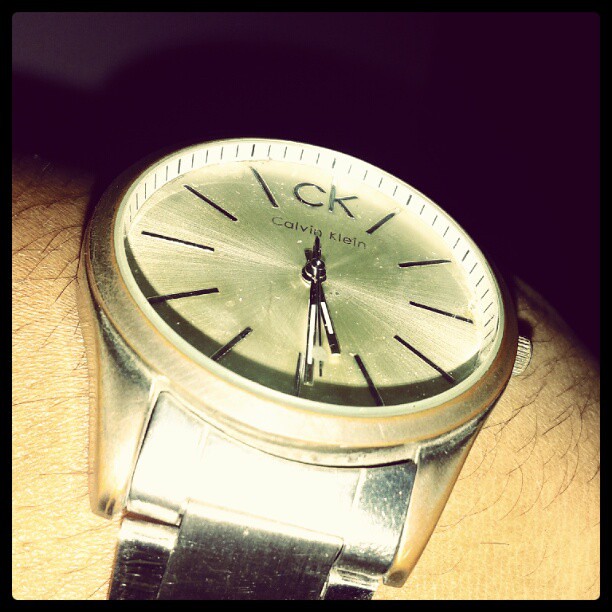This close-up, square color photograph captures the wrist of a person wearing a Calvin Klein wristwatch. The shot, taken at an angle and illuminated by what appears to be a cell phone camera flash, focuses on the watch face that is goldish and features visible wear with white spots around the edges. The watch, which is mounted on a person's wrist with coarse, dense black hairs, has a black leather wristband. The face of the watch is analog with no numbers, only silver vertical lines to mark the hours and finer vertical lines along the inner perimeter for the minutes. Prominently at the 12 o'clock position is the CK logo, with the brand name "Calvin Klein" written underneath. The watch hands, also in a reflective stainless steel, indicate that the time is approximately 5:30. The watch body and winding dial are silvery, contrasting with the worn, golden watch face, and the photograph gives a sense of the watch being quite old.